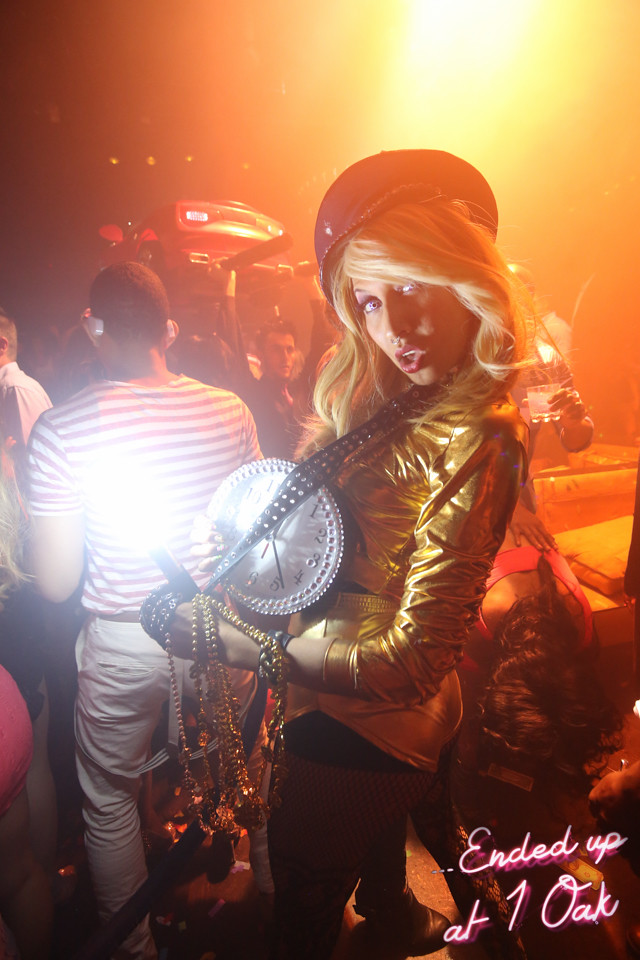A captivating image from inside a nightclub, presumably named One Oak, features a striking woman at its center. She has long, blonde hair cascading from under a black hat, which sits slightly askew on her head. Her eyes are wide, lips parted as if she's in mid-sentence, accentuating her dynamic presence. She wears a shiny, form-fitting golden top paired with very short gold shorts over black tights. Draped across her chest by a black strap, she clutches a distinctive silver clock, reminiscent of Flava Flav's iconic style. In her other hand, she holds several beaded necklaces and what appears to be a black stick emitting light, perhaps a small flashlight. The background is bustling with energy; blurry yellow lights and indistinct figures, including a man with dark, short hair in a red and white striped shirt, add to the frenzied atmosphere. Two men grip black bars above the crowd, suggesting a lively dance floor scene. The bottom right corner of the image bears the text, "Ended up at One Oak," grounding this energetic vignette in its vibrant setting.